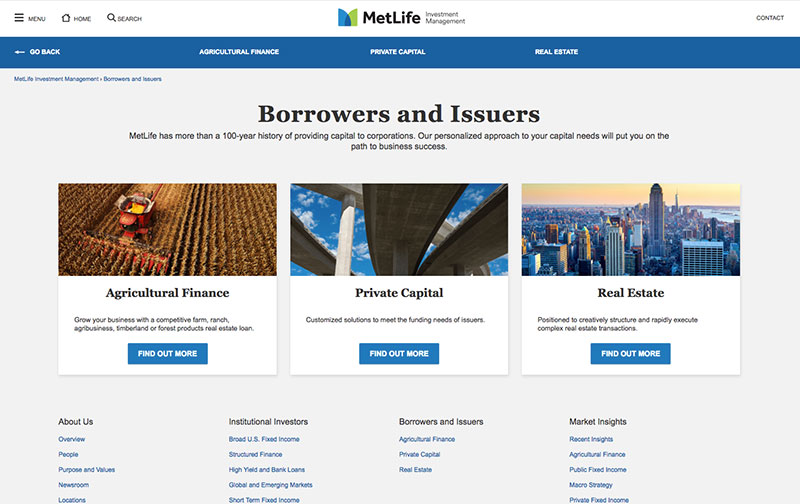The image contains detailed promotional content for MetLife's investment mentoring and financial services, set against a white and gray background. The top portion highlights MetLife's extensive history, over a century, in managing capital corporations and provides reassurance with a personalized approach to capital needs leading to business success. The upper section features a square labeled "Agricultural Finance," suggesting MetLife supports competitive farming, ranching, timberland, and real estate through tailored business proposals and loans.

In the middle section, a larger rectangle titled "Private Capital" outlines three customized solutions to meet funding needs, emphasizing MetLife's capability to creatively structure and execute complex real estate transactions. This section also depicts numerous buildings, underscoring their extensive real estate services. Another rectangle prompts viewers to find out more about the company, hinting at services for institutional investors including people, purpose, values, needs, and multiple locations.

An orange box in this area emphasizes MetLife's offerings in fixed income, short-term finance, high yield, bank loans, and global and emerging markets. It also revisits services in agricultural finance, private capital, and real estate, while mentioning insights in market trends, macro strategy, and public and private fixed income.

Overall, the image is designed to illustrate MetLife's vast network and expertise in various financial services and investment solutions, using detailed segments to convey its comprehensive approach to supporting business growth and financial stability.